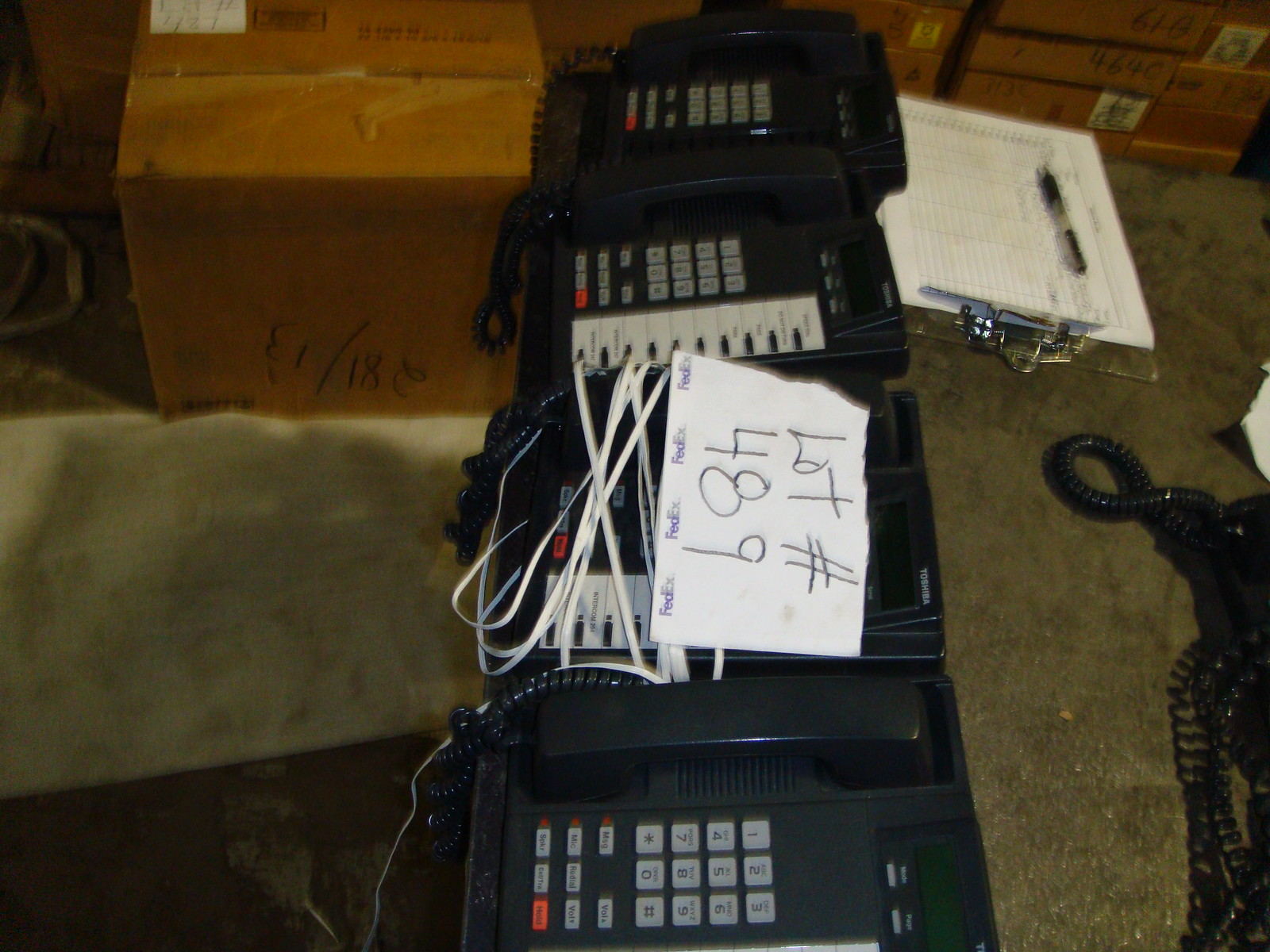The photograph presents an indoor scene with four used, black office phones aligned vertically from the bottom to the top of the image. The phones are identical in model, featuring grey keypads and an orange button, with headsets facing upwards. A white piece of paper is attached to the central phone, marked in black ink with "lot number" and "489," followed by the word "FedEx" printed multiple times along the bottom. The arrangement suggests these phones might be up for auction. Scattered around are various items: in the upper right, a rectangular cardboard box with partially visible numbers; below it, part of a desk with a clipboard, the clip pointing downward and a pen placed vertically; and on the lower left, what appears to be a dirty, white cloth with brown smudges. Additionally, several cords from other phones are partially visible on the right side. The background and the surface, possibly concrete, add to the busy, cluttered atmosphere of what seems to be a storage or auction preparation area.